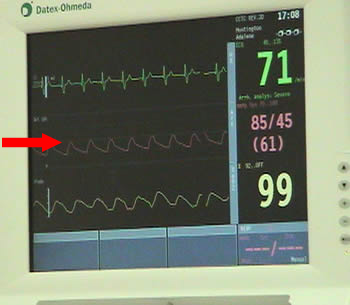This is a detailed photograph of a vital signs monitor, predominantly showcasing its screen, which occupies most of the frame except for the narrow plastic framework around the edges. The screen, primarily black, belongs to a Datex Ohmeda brand monitor, as indicated by the logo at the top. The display features three horizontal readouts: the top line displays a heart rate with the number "71" on the right-hand side; the middle line shows a blood pressure reading of "85/45," with "61" in parentheses; and the bottom line indicates an oxygen saturation level of "99." A red arrow points to the center readout. Various control buttons, including up, down, plus, and minus, are visible on the machine's light gray surrounding framework. Additionally, the screen includes a time stamp and possibly a date.